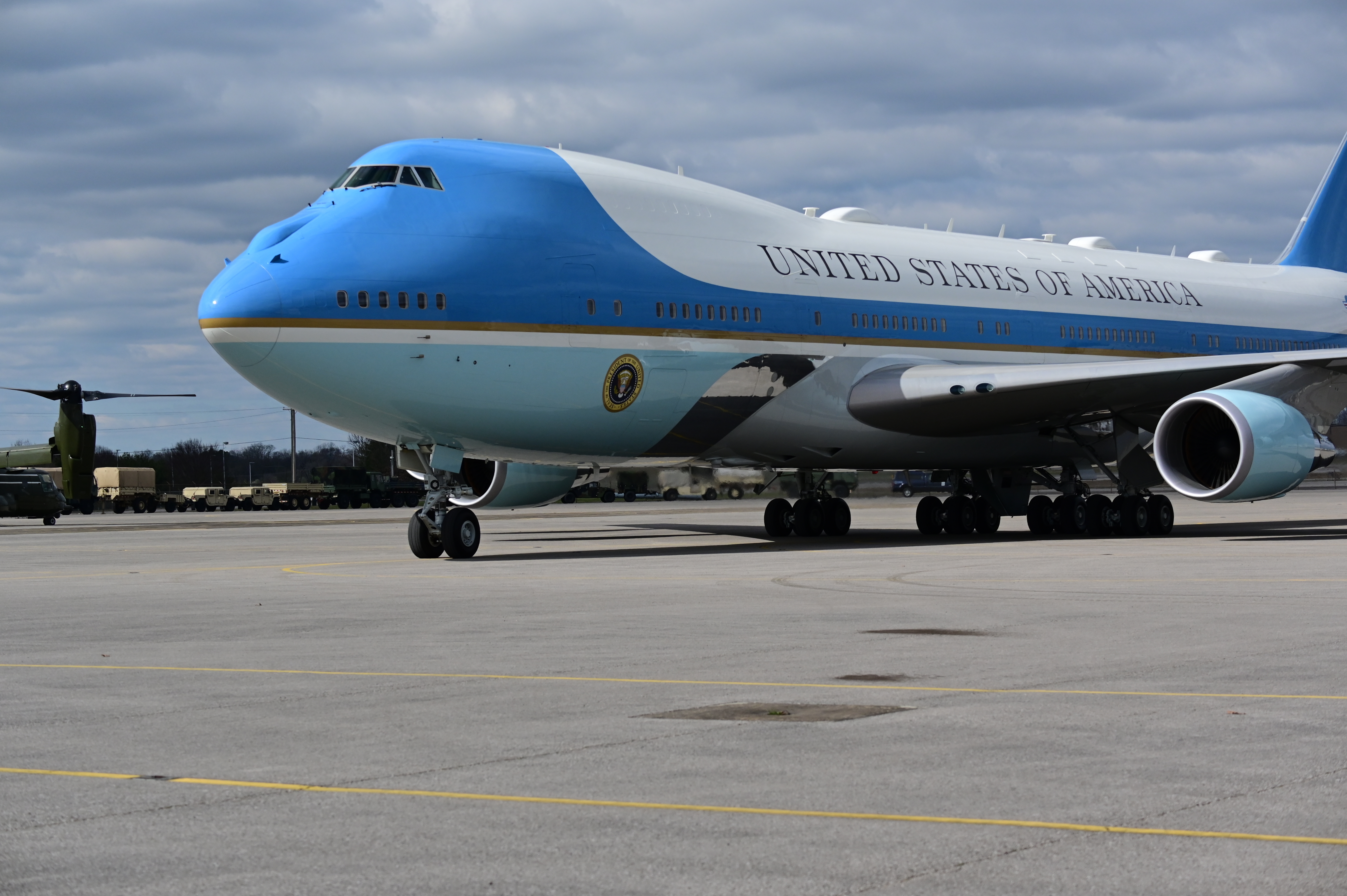In this detailed image of Air Force One, the distinctive Boeing 747 jetliner, the plane is seen parked on a runway under a mostly cloudy, gray, and white sky. The upper section of the aircraft is white, with "United States of America" prominently displayed across it in bold letters. Just below this, the top section is marked by a blue field that extends over the pilot's quarters. Beneath the blue field is a gold band followed by a white stripe. The lower portion of the plane’s body features a light blue color.

The imposing structure of the plane includes the visible front section displaying the presidential seal near the nose, but not quite to the cockpit. The image captures the aircraft stationary with its landing gear down, clearly showing the tires and the bottoms of the multiple wheels—two in the front and four on each of the main landing gears. The plane's point of view is directed towards the left side of the photo.

In addition, one of the wings and the engine situated below the wing are clearly visible. The partially visible tail at the rear of the plane is also colored blue. On the far left edge of the photo, the propeller and wing of an Osprey aircraft are seen, amidst a background that includes tan-colored Army vehicles. The runway itself features yellow stripes running across horizontally, enhancing the scene's detailed setting.